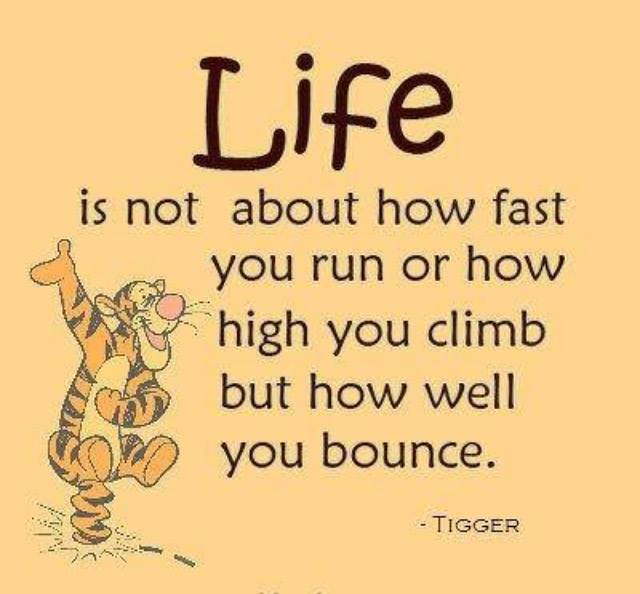This captivating poster features an inspirational quote set against a vibrant background that transitions from yellow to a light orange hue. Dominating the top of the poster is the word "LIFE" in bold black letters, notably larger and in a different font than the rest of the text. The full quote reads, "Life is not about how fast you run or how high you climb, but how well you bounce." The words are in black, with "LIFE" standing out prominently.

At the bottom of the poster, the quote is attributed to "TIGGER," written in all capital letters. On the left side, towards the bottom, there is a colorful, animated image of Tigger. He is depicted with his signature black and orange stripes, a pink nose, and a pink mouth, joyfully bouncing on his tail. Tigger's raised paw and big smile add a cheerful touch, reinforcing the message of resilience and optimism. The contrasting shades of orange between Tigger and the background make him stand out, further enhancing the visual appeal of this motivational poster.